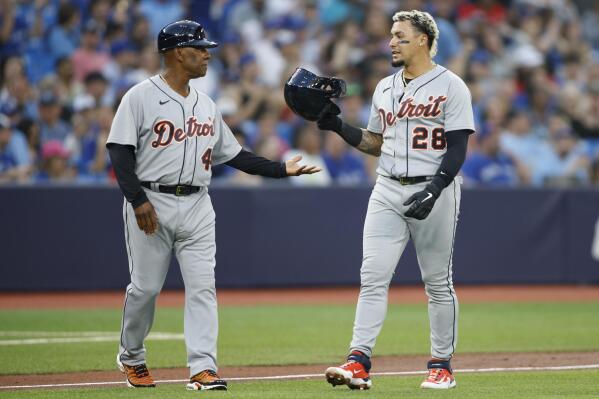This photograph captures an action moment from a professional Major League Baseball game, featuring two players on the field in Detroit uniforms. The player on the left, who might be a coach, sports the number 4 on his jersey and has brown skin. He is reaching out his hand towards the player on the right, who wears the number 28 and has short blonde hair, lighter skin, and is holding his batting helmet in his hand. Both players are wearing long sleeved shirts under their jerseys, as well as red, white, and black shoes. The scene is set inside the infield, with a blurry background showcasing a crowd of fans mostly clad in blue shirts, contained by a blue mat.